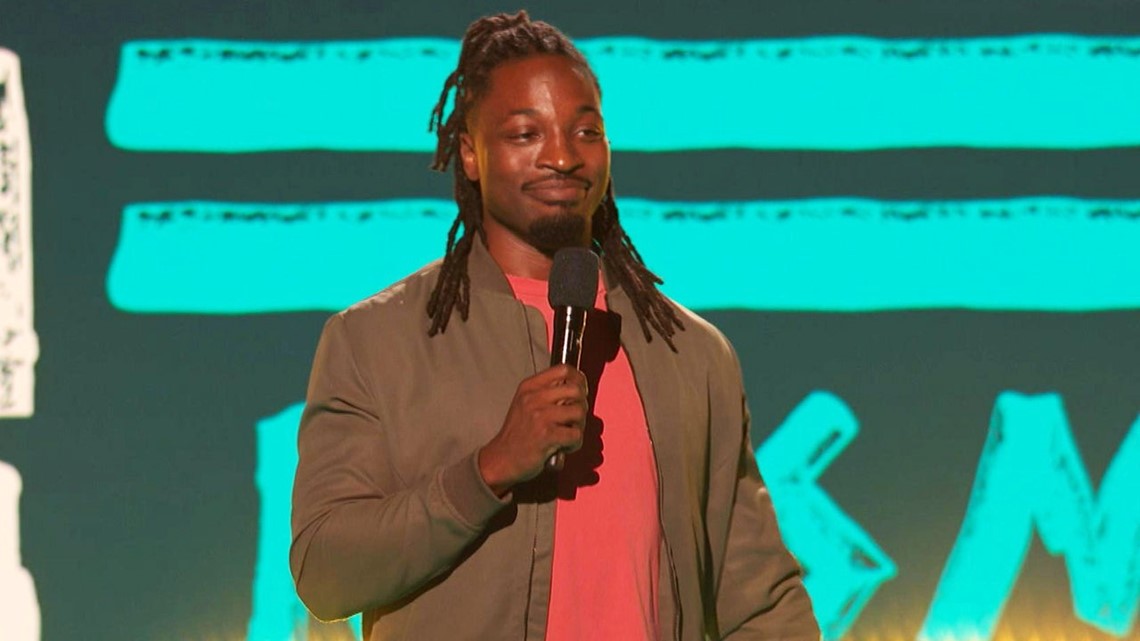The photograph captures a black man standing on a stage, seen from the waist up. He has dark skin and shoulder-length dreadlocks, with the front part pulled back into a high ponytail. His facial features include a triangular nose, slightly small ears, large lips, a thin mustache trimmed into a line, and a small circular beard on his chin. He is smiling and appears to be addressing an audience, holding a microphone at chin level with his right hand. He is dressed in a brown zip-up jacket, which has a waterproof appearance, over an orange shirt. The backdrop behind him is green with two horizontal turquoise stripes and partial turquoise letters, obscured by his presence on stage. The photograph, taken indoors, suggests the man is engaged in a presentation or performance.